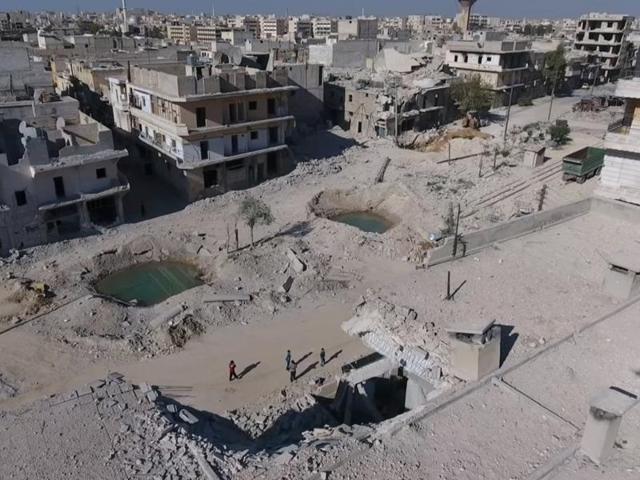In this aerial shot of a construction site, the area is dominated by sand and rubble, suggesting recent upheaval or excavation. Central to the image is a large rectangular foundation with a significant hole, surrounded by four individuals seemingly poised to work. Adjacent to this scene lie two water-filled craters, separated by a small tree. The light gray ground gives the impression of either dust or debris. Beyond this central activity, the background is filled with numerous whitish-gray buildings, one notably appearing dilapidated with a crumbling roof. Despite the apparent destruction, the skyline at the top of the image is serene, marked by a strip of blue sky stretching across the photograph.